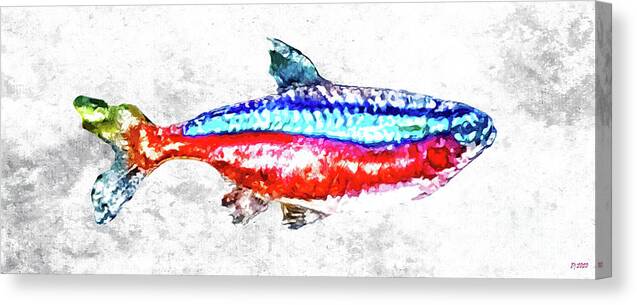This image showcases a vibrant, multi-colored fish depicted in a graphic design style on a three-dimensional, rectangular canvas that is approximately an inch thick. The background of the canvas is predominantly white, interspersed with patchy gray areas that give it a marble-like texture. The fish itself is not realistic but rather an artistic interpretation, featuring an array of bright and shimmering colors including electric blue, turquoise, red, pink, green, and silver, with streaks and glints of white and gold adding to its iridescence. The fish, which appears to be swimming towards the right side of the canvas, has a serious expression with its blue eye open and a closed mouth. Its body is striped with the fins and tail exhibiting various colors; the top fin is blue and white, the body transitions from white to dark blue to red on its underbelly, and the tail displays hues of green, red, light blue, and dark blue streaks. The entire piece is angled to the side, enhancing its three-dimensional effect as a wall hanging.